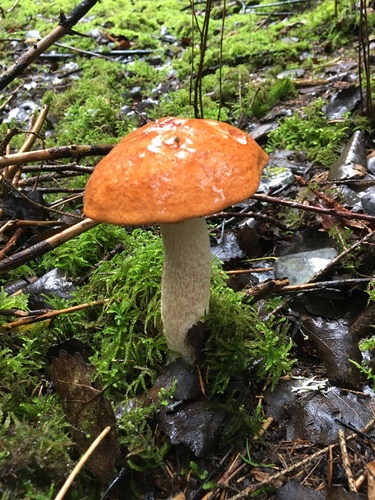In this detailed portrait-oriented color photograph, a striking Leccinum arantiacum mushroom stands as the focal point, emerging prominently from the lush, green forest floor. The forested hillside setting is filled with low-growing plant life and moss, alongside scattered twigs, sticks, and fallen tree limbs, hinting at the damp, earthy environment. The mushroom proudly reaches approximately three to four inches above the ground on a tall, cream-colored stalk, crowned by a distinct umbrella-shaped cap that is a vivid orange adorned with white speckles. The earthy forest floor displays a hint of wetness, possibly with some small watery patches, enhancing the textured natural scenery and emphasizing the photographic representational realism style of the image.